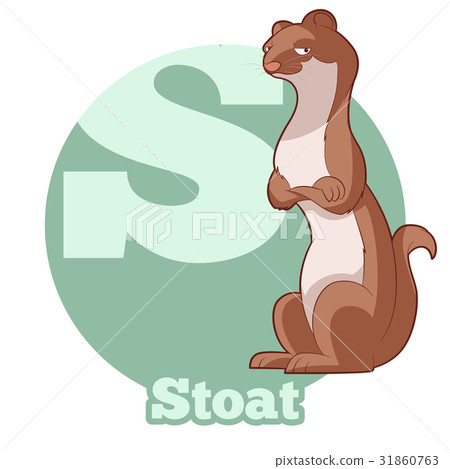The image is a detailed animated depiction of a stoat standing upright on its hind legs. The stoat, with a dark brown back and face, contrasts against its light grey and white underbelly and lower face. It has a semi-long brown tail and a distinct pink nose. The stoat's arms are crossed, and it wears an irritated, almost angry expression while looking directly at the viewer with both eyes visible. The backdrop features a large light mint-green circle encompassing an even lighter mint-green letter 'S' at the top. At the bottom of the circle, the word "STOAT" is spelled out in capital bubble letters. Additionally, there is an icon with the name "Pixta" situated centrally in the image.